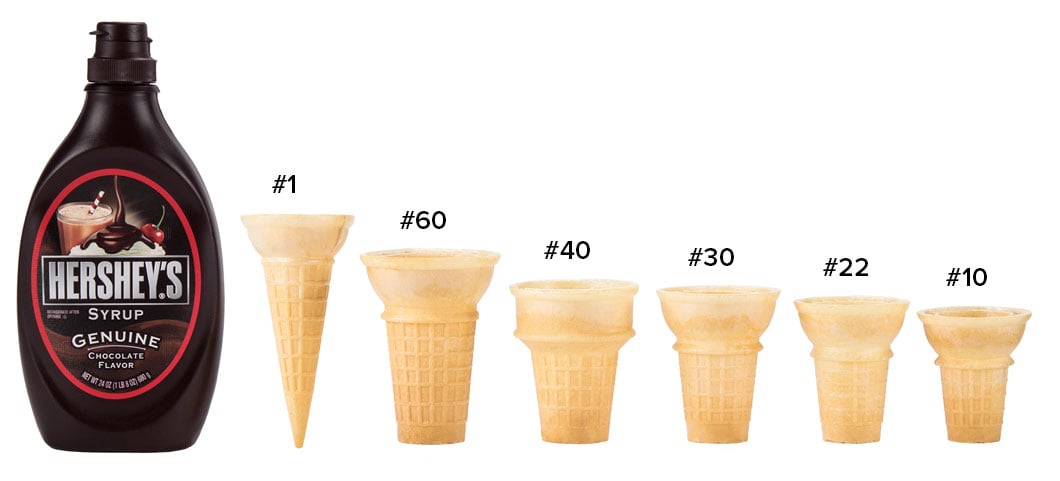This horizontal advertisement showcases a featured image of Hershey's Syrup on the far left. The iconic dark brown bottle, fitted with a bump cap, prominently displays the Hershey's label in an oval, vertically oriented shape. A stream of rich, chocolate syrup is illustrated pouring generously onto a scoop of ice cream, crowned with a vibrant cherry. The rectangular section of the label reads "Hershey's," followed by "Syrup" and "Genuine Chocolate Flavor" beneath.

Adjacent to the syrup bottle, a variety of yellow, waffle-bottomed ice cream cones are displayed in a neat row. Each cone is distinctly numbered: Number 1, Number 60, Number 40, Number 30, Number 22, and Number 10. The pointed cone, denoted as Number 1, leads the sequence. All cones are presented against a clean, white background, emphasizing their details and the standout quality of Hershey’s Syrup. This detailed and visually appealing layout makes a compelling case for Hershey’s Syrup as the perfect companion for a delicious ice cream treat.